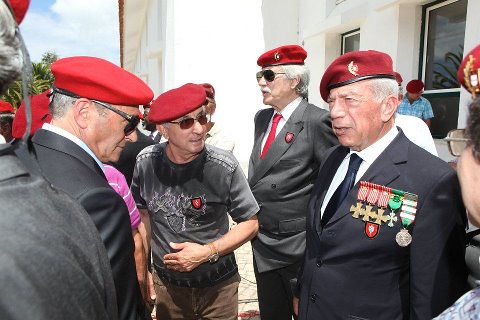This detailed color photograph captures a gathering of predominantly older men, who appear to be veterans, identified by their military-style crimson red berets and various medals. The central figure, standing to the right and facing slightly left, is notably dressed in a navy suit jacket, white shirt, and dark tie, with several bronze crosses pinned on the left breast pocket area, indicative of military honors. These men, mostly in their 50s, 60s, or older, are engaged in conversation. The setting is outdoors, beneath a sky of white clouds and patches of blue. In the background, a white or sand-colored stone building with vertically aligned, black smoke-glassed windows is visible. Additionally, some women and palm trees are discernible in the far backdrop, further suggesting a military reunion or commemorative event.